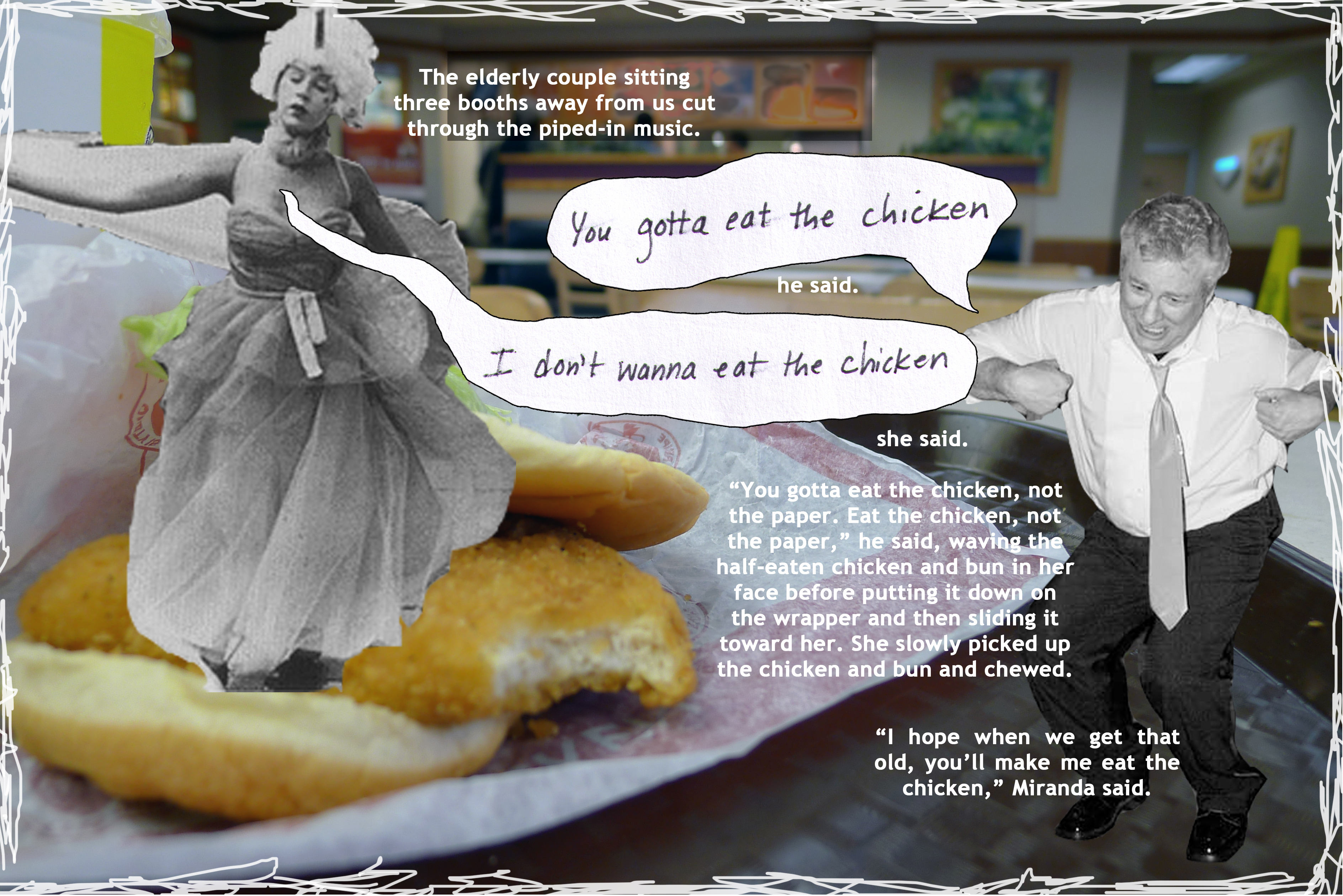This image showcases a cleverly composited meme created in Photoshop, set in what resembles a college student union cafeteria. The left side of the image prominently features a close-up of a fried, breaded chicken sandwich partially wrapped. Blurry artwork is visible on the background wall, accompanied by long dining tables, adding to the bustling cafeteria atmosphere.

The image is framed with an electronic-looking border, characterized by a rough, white, scribbled line. Within this frame are two striking black-and-white photographs: On the left is a woman donned in a long, flowy, theatrical dress paired with a voluminous wig, a beauty mark accentuating the area below her left eye. To the right is a man performing the chicken dance, dressed in a white shirt and long tie, with his hands tucked into his armpits.

Accompanying these visuals is text, which narrates a humorous story about an elderly couple seated three booths away from the viewer, loudly cutting through the piped-in background music. The woman exclaims, "I don't want to eat the chicken," encapsulated in a word bubble, while the man, with a determined expression and a word bubble of his own, responds, "You got to eat the chicken." Additional text below continues this playful exchange, elaborating on the mini-drama about the woman's reluctance and the man's insistence regarding the chicken sandwich.